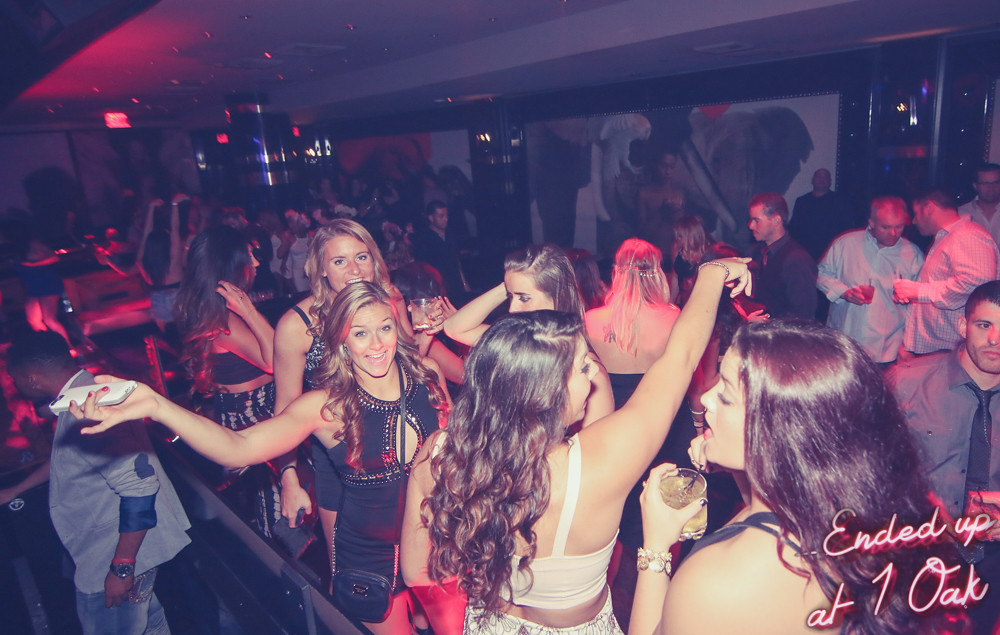The photograph captures a lively night at One Oak nightclub, featuring a vibrant and crowded dance scene. In the foreground, several young women dominate the frame, exuding energy as they dance, smile, and wave. At the bottom center and right, two women with their backs to the camera are caught mid-dance. The woman on the bottom right, with brunette hair and dressed in black, holds a yellow-tinted alcoholic drink in a plain glass, seemingly shouting towards the center of the frame. 

To her left, another woman faces the crowd, sporting long brunette hair curling at the ends and a white tank top. In the left center, a blonde woman in a black dress smiles directly at the camera, extending her hand that clutches a white cell phone while a black purse strap rests on her shoulder. Behind her stands another blonde woman, also smiling at the camera, holding a similar yellow drink in a small glass. 

The backdrop reveals a busy dance floor teeming with party-goers, lit by a mix of red and white lights emanating from the DJ's platform and overhead strobe lights. The club's ceiling is visible, featuring standard white tiles and air ducts. A large, partially obscured mural decorates the back wall. Splashed across the lower right corner of the photo in cursive neon print is the phrase "Ended up at One Oak," adding a final touch to this dynamic scene of late-night revelry.